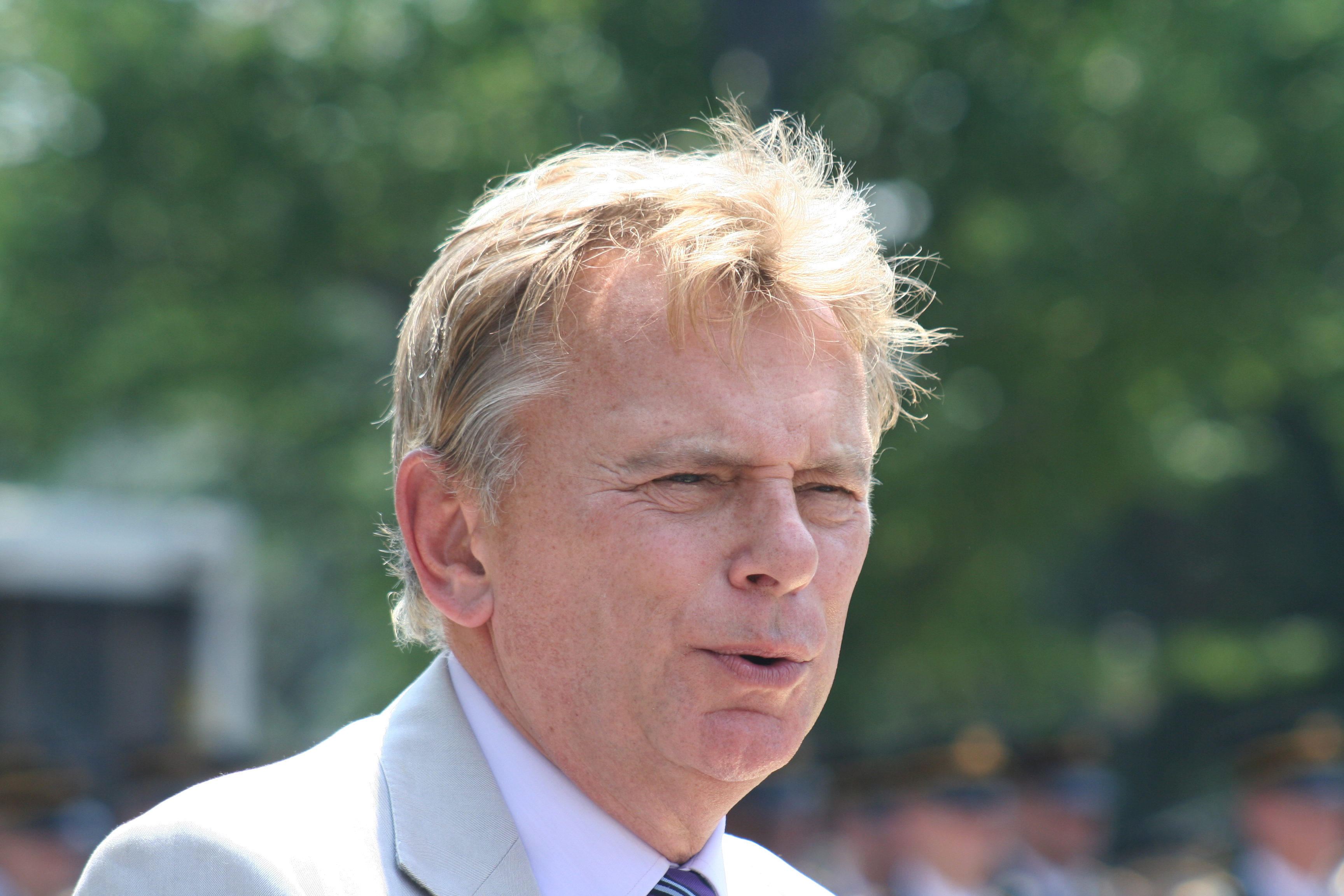In this outdoor photograph likely taken at an event or press conference, an older gentleman who bears a striking resemblance to Pat Sajak is the central figure. He appears to be in his 50s to early 60s, with a pale complexion and of Caucasian descent. His blonde hair, which is beginning to gray, is slightly messy, likely tousled by the wind, and not held down by gel or pomade. He is captured in mid-sentence, his mouth forming a word, and is squinting, possibly due to bright sunlight that is casting a glare on his face.

Sajak is dressed in a very light gray or beige-colored jacket or blazer, paired with a white button-down shirt. His necktie, which is partially visible, seems to be dark blue with light blue stripes, though it is mostly cut off at the bottom of the image. He has distinct wrinkles around his eyes, highlighting his age.

The background is quite blurry but gives the impression of an outdoor setting, featuring trees and possibly a building on the left side. Vaguely identifiable in the lower right corner are figures resembling military or police personnel standing in a row. Despite the lack of clarity in the background, the scene suggests a formal or official occasion, with the focus firmly on Sajak as he addresses someone or something unseen in the photograph.